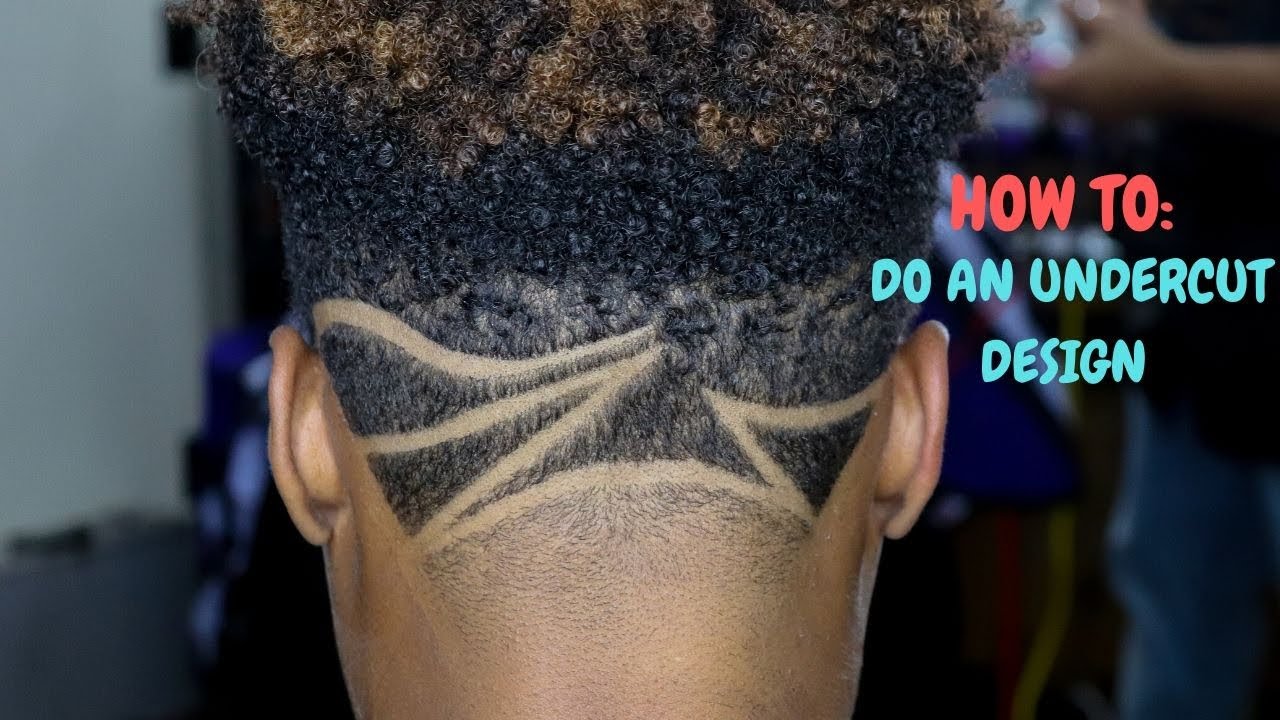The photograph, taken presumably in a barbershop, captures the intricate design razored into the back of an African-American individual's freshly cut hair. The head, centered in the frame, showcases a meticulous undercut design featuring a variety of colors: black, brown, yellowish gold, red, a little blue, and bluish green, almost like aqua. Positioned in the middle towards the top, the design is surrounded by the person's short hair, with their ears visible on either side. The background is a blurry blue, heightening the focus on the hair design. Off to the right in a pink hue, the text reads "How to: Do an undercut design" in blue font underneath, suggesting the image is part of a tutorial or instructional content. The setting and blurred indistinct shapes hint at the busy environment of a barbershop.